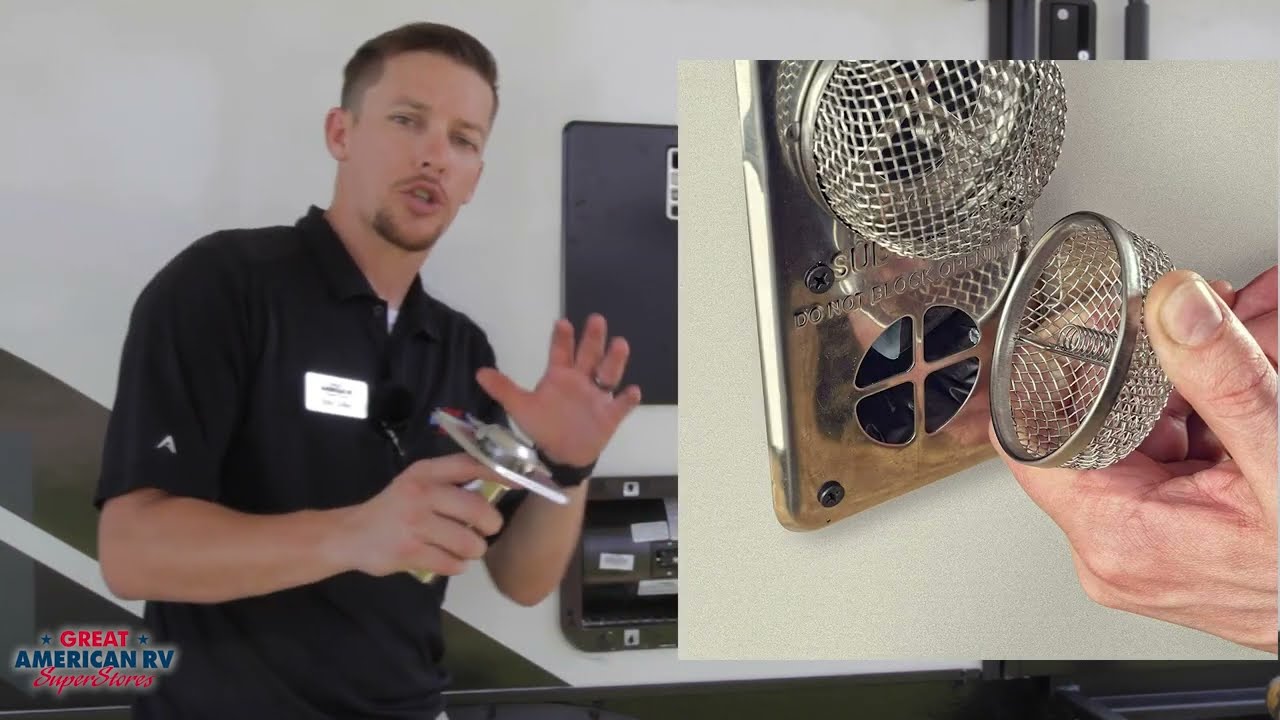This image appears to be a screenshot from a video, possibly an advertisement or tutorial from Great American RV Superstores. The focal point is a man who seems to be a professional, perhaps a mechanic or electrician, evidenced by his black short-sleeved shirt, white name tag, and company logo. He has short brown hair, a beard, and a mustache. The text "Great American RV Superstores" is prominently displayed in the lower left corner of the screen. Behind the man is a white wall featuring some indistinct black machinery. In his right hand, he holds a metal tool. On the right side of the image, a detailed insert shows this same man using a chrome-like, circular metal device, which resembles a vent or a similar RV part. His hand is seen installing this device onto the side of an RV, emphasizing his demonstration of the product's application and function.